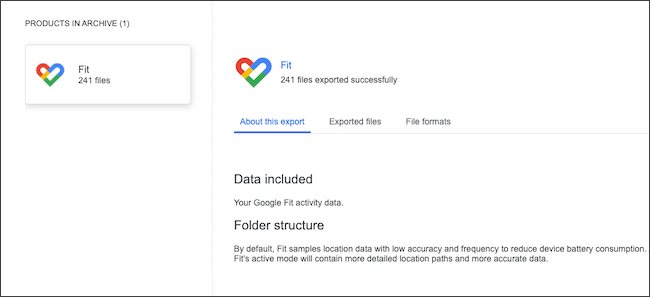Screenshot of a Google Fit Activity Data Export

This screenshot displays a Google Fit activity data export, showcased prominently by the Google Fit app's interface. In the upper left corner, there is the recognizable Google Fit logo, a heart shape featuring Google’s signature multicolor scheme. Adjacent to the logo, a button is highlighted, indicating its selection.

The primary content area is marked by plain, dark blue text on a white background, detailing information about the exported data. The text states "Products in Archive and Fit" near the top. Below, the header announces that 241 files were successfully exported. These files likely represent daily workouts or related fitness data.

Highlighted in the section titled "About this export," it mentions that the data includes your Google Fit activity statistics. A notable detail indicates that, by default, Google Fit samples location data with low accuracy and frequency to conserve battery life. However, in active mode, the app collects more detailed and accurate location paths.

Overall, the screenshot efficiently presents an overview of the exported fitness data from the Google Fit app, emphasizing the balance between data accuracy and device battery conservation.